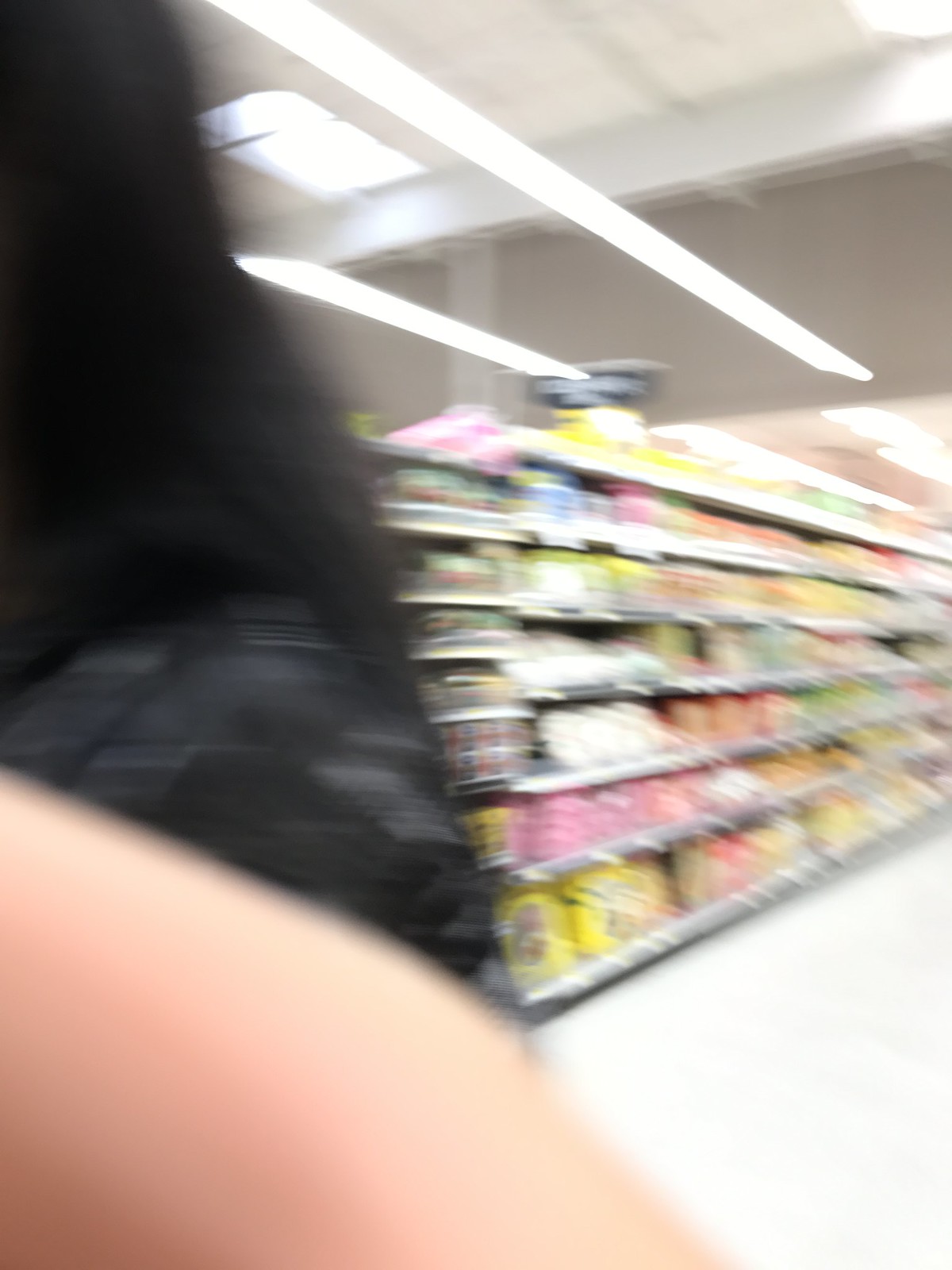In this dynamic photograph taken inside a grocery store, the background is lined with shelves stocked with products displaying a vibrant palette of colors, including yellows, reds, whites, and greens. The motion blur in the image renders the items indistinct, blending them into a colorful haze. In the lower left corner, a portion of a person is visible; their hand, likely holding the camera, shows a glimpse of skin tone. Their shoulder, clad in a dark black and gray shirt, and their long, dark black hair extending to the shoulder area, can also be seen. Overhead, a white ceiling adorned with a prominently featured fluorescent light hangs low, illuminating the scene.